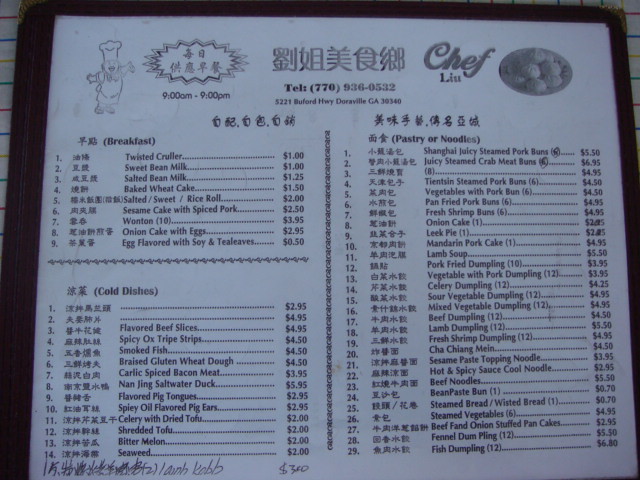Caption: 

Photograph of a menu from Chef Liu's restaurant, located in Georgia. The menu is printed on white paper using grey and black ink, encased in a protective plastic cover, and presented within an elegant leather folder. The menu is primarily in Chinese with English translations next to each item for easier navigation. The breakfast section features 9 items, there are 15 cold dishes, and an extensive selection of 29 pastry and noodle dishes. Notably, "lamb kebab" has been handwritten in both Chinese and English, indicating a specialty addition not originally printed on the menu.